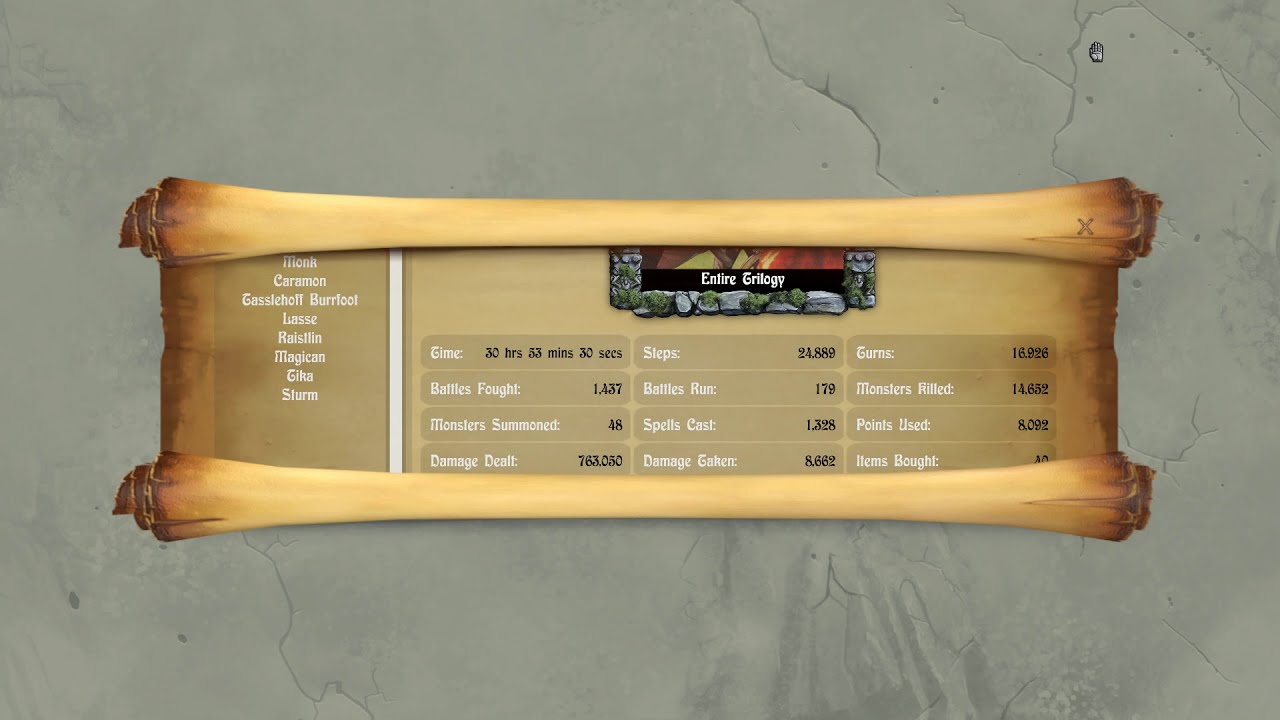The image features a game score displayed on a digital dashboard designed to resemble an ancient paper scroll. The scroll has rolled up edges at the top and bottom and is framed with a cracked stone border, giving it an aged look. Within the scroll, there is text positioned on the left side listing the names: Monk, Karamon, Tasselhoff, Burfoot, Lassli, Raistlin, Machikon, Chica, and Sturm, all in white text. 

The main section in the center of the scroll is divided into three columns detailing various game statistics: time played (30 hours, 53 minutes, 30 seconds), battles fought (1437), monsters summoned (48), damage dealt (763,050), steps taken (24,889), battles run (179), spells cast (1328), damage taken (8662), turns played (16,926), monsters killed (14,632), points used (8092), and items bought (10). 

The dashboard itself is set against a stone background, possibly mimicking a kitchen counter in appearance, with a small armored hand appearing at the top right corner, near a white 'X' mark.

This robust scoreboard captures various intricate details of the player’s journey and achievements within the game, providing a comprehensive overview of their progress.